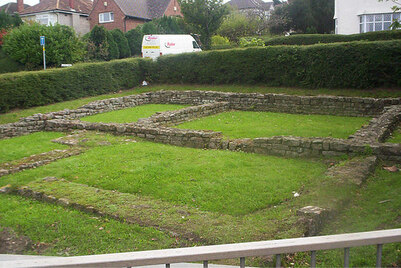Taken from a wooden balcony with thin slats and a simple armrest, the image depicts a meticulously maintained yard that resembles a historical site, possibly a backyard or a park. The lawn is freshly cut and bordered by dark green hedges. In the middle of the yard lies a large, square area of grass, with remnants of a stone structure—likely the crumbling base of an old building, made of sizable gray stones. The stones primarily remain piled up in the back area of the structure. In the background, a well-trimmed line of hedges stretches across the image, framing a residential neighborhood where several brick-faced and red brick houses are visible. Among these houses, a modern white delivery van can be seen driving past. The scene suggests a serene setting that blends historical and contemporary elements.